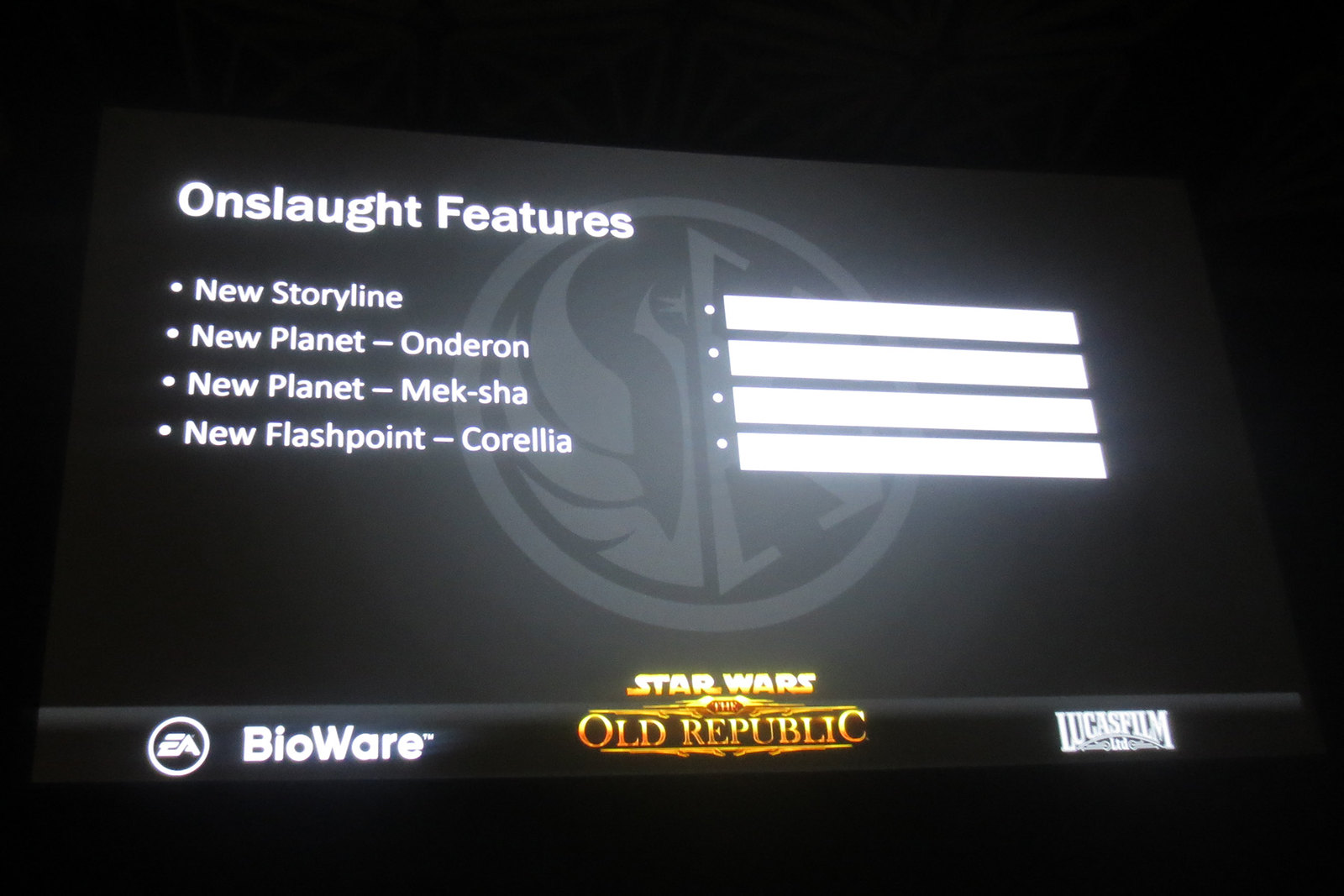The image is a digital photograph taken at a conference presentation for a new video game update, specifically for "Star Wars: The Old Republic." The scene is centered around a large projector screen set against a black or dark grey background. At the top center of the screen, there is an emblem resembling a shield or a winged eagle, possibly representing the Imperial Force from Star Wars. The primary text on the screen is in white font and reads "Onslaught Features," followed by several bullet points detailing new additions to the game: "New Storyline," "New Planet: Onderon," "New Planet: Meksha," and "New Flashpoint: Corellia." To the right of these points are four more bullet points with white borders, likely indicating future reveals. At the bottom of the screen, logos for EA BioWare, Star Wars: The Old Republic (in a distinct gold font), and Lucasfilm Limited (in white) are prominently displayed. The colors in the image are predominantly black, white, and gold, contributing to the formal and high-tech feel of the presentation.